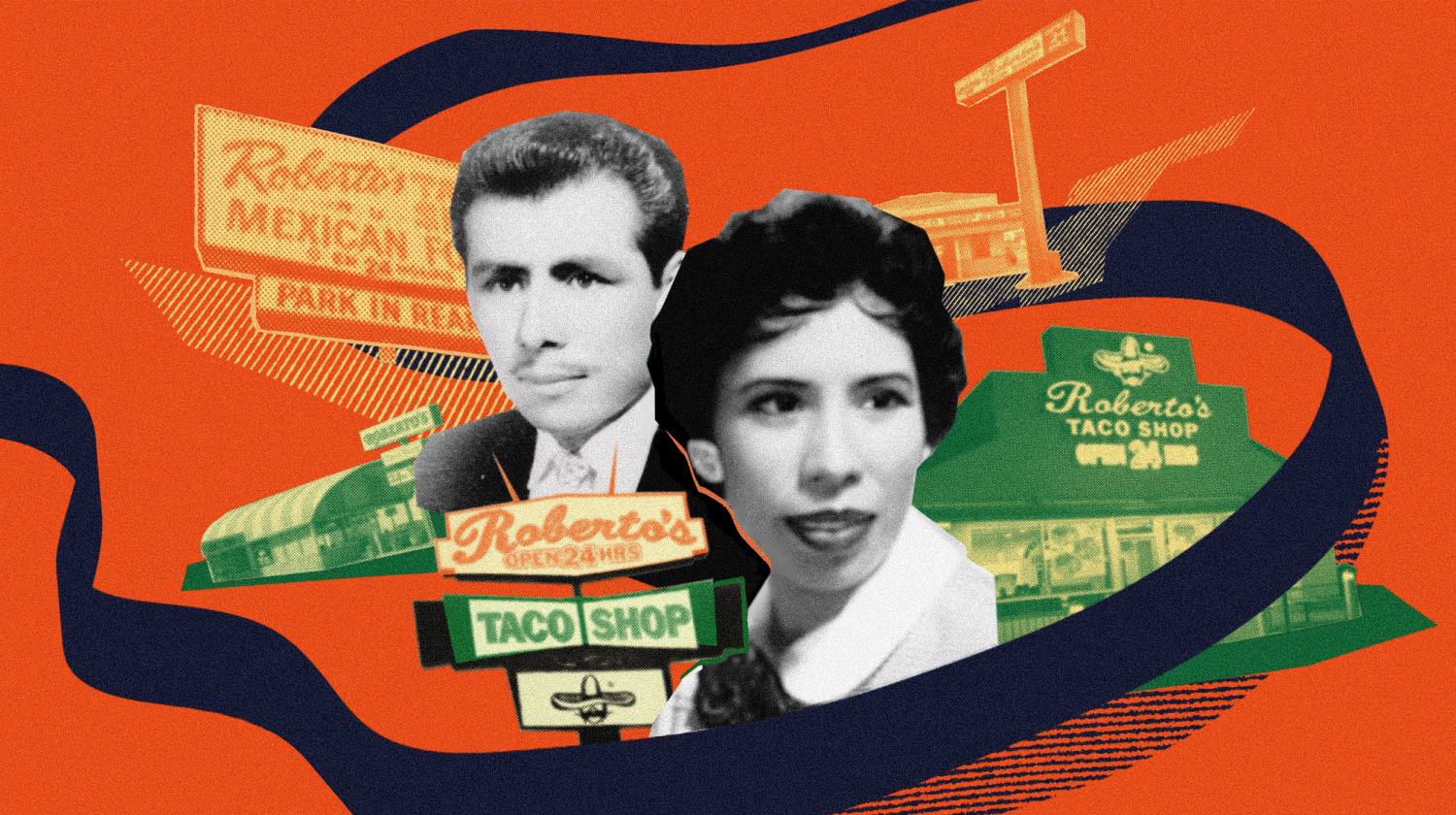The image is a vintage-style collage celebrating Roberto's Mexican Food, perhaps from the 1950s or 1960s, featuring prominently on an orange-red background with a black ribbon running across it. The central focus is on two black-and-white portraits of the establishment's founders. On the back left is the man who runs the operation, characterized by his prominent eyebrow bridges, slight mustache, and short black hair. Below his chest portrait, there's a sign that reads "Roberto's Open 24 Hours Taco Shop." On the right is the woman co-owner, depicted with short black hair, lipstick, earrings, and possibly a white coat. Additionally, various depictions of the taco shop building itself appear, floating around the image, with "Roberto's Taco Shop" inscribed in different colors. This collage visually narrates the legacy and founders of Roberto's Taco Shop.